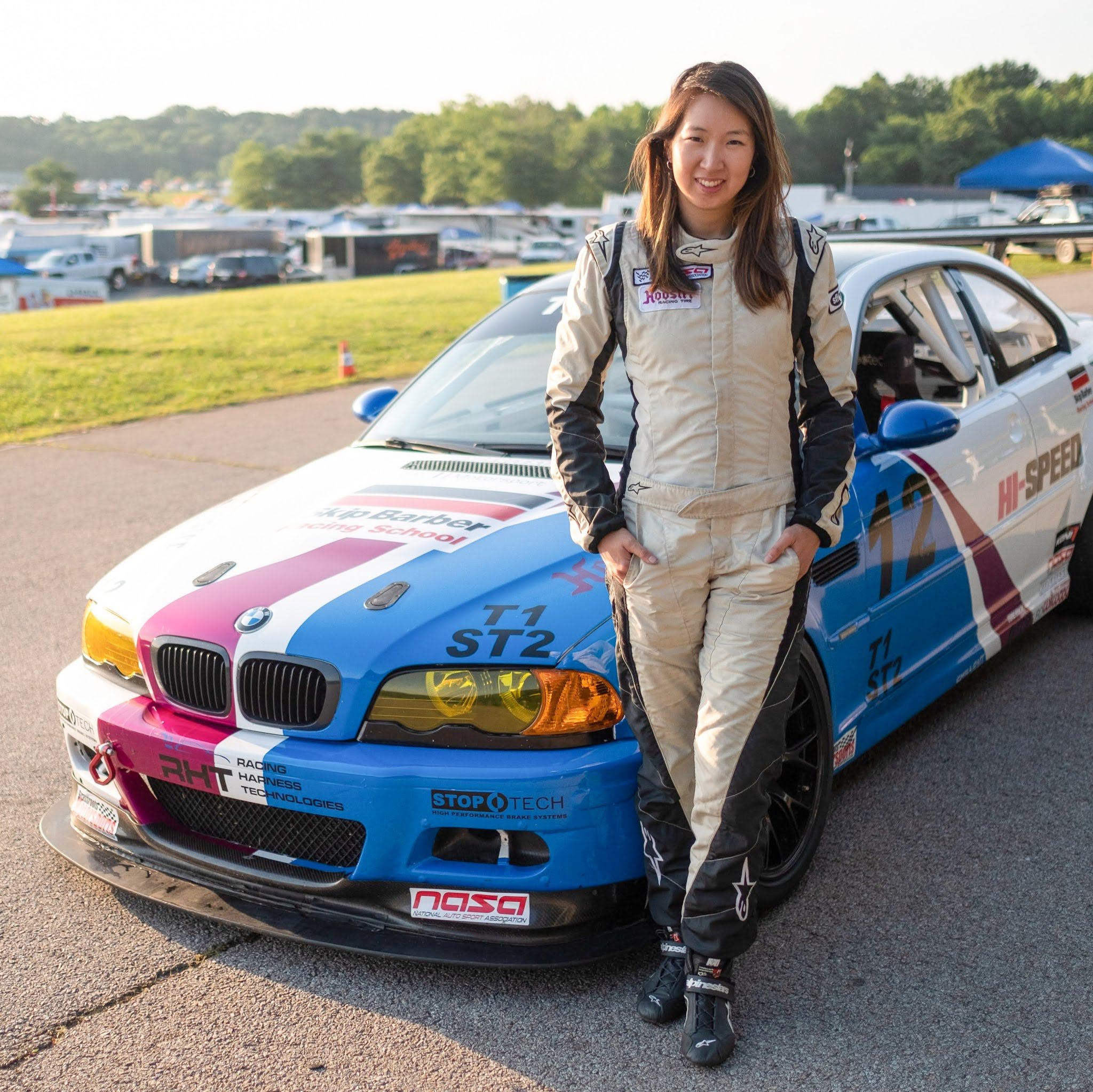In this color photograph, presented in landscape orientation, an Asian woman named Christina Lamb stands confidently in front of a race car. She has long, light brown hair, suggesting it might be dyed, as natural Asian hair is typically black. Christina wears a beige racing uniform accented with black stripes on the sleeves and pants. She is smiling warmly at the viewer, her stance casual with legs crossed and hands in her hip pockets. 

The race car behind her, potentially a BMW, boasts a white body with accents of red, blue, and magenta, adorned with various sponsor logos including "NASA" (National Auto Sport Association) and "RHT" (Racing Harness and Technologies). The car also displays the number 12 in black graphics. The photograph is taken during the daytime, as evidenced by the multiple non-racing vehicles and dark green trees visible in the distant background. The style of the image is grounded in photographic realism, capturing the scene with vivid detail.